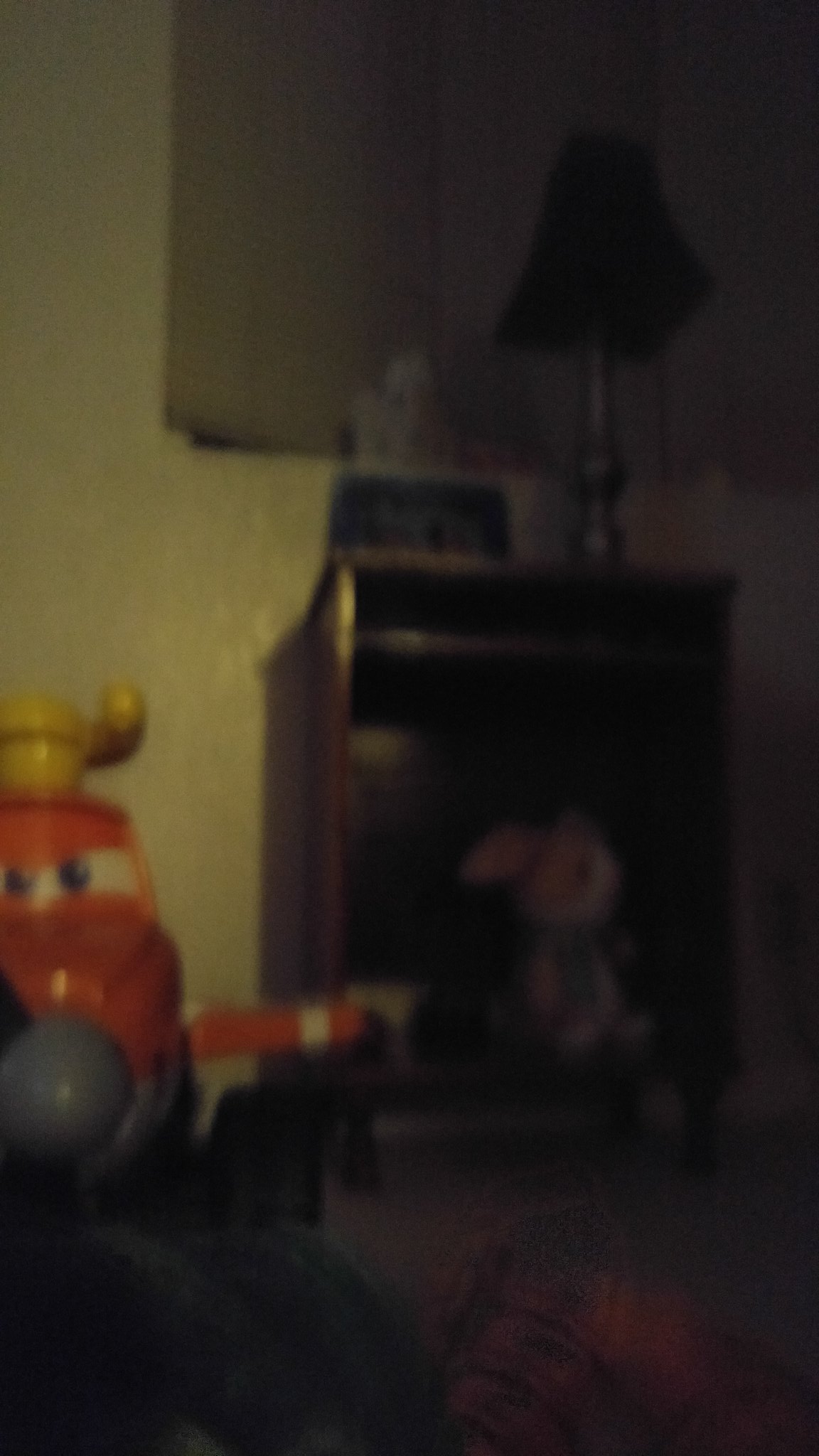The image depicts a dimly lit child's bedroom with some scattered items illuminated by light from behind the left side. Central to the scene is a nightstand or small dresser with two compartments. On the top surface of the nightstand, there is a digital clock or picture frame with a bluish tint and a lamp with a greenish lampshade and a metal base. Behind the nightstand are gray curtains. In the bottom compartment of the nightstand, a pink stuffed bunny is visible. The floor near the nightstand is dark, adorned with a brown item resembling a baseball mitt. To the left of the nightstand, an orange and red ride-on toy with eyes and a yellow steering component, reminiscent of a character from Pixar's Cars movies, stands out. The walls of the room are a beige color.